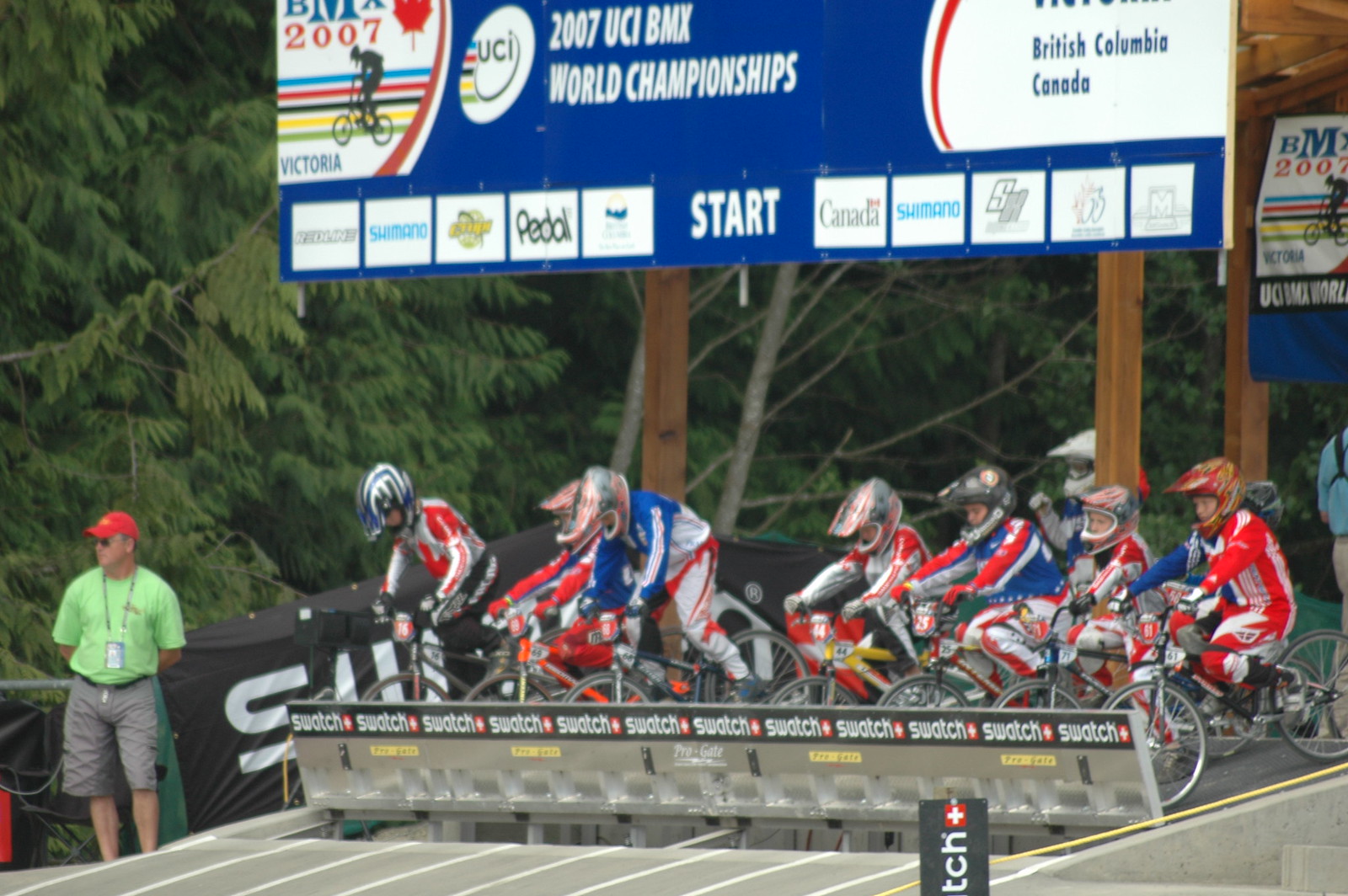In this detailed photograph of the 2007 UCI BMX World Championships, we see an intense moment at the starting gate. Eight young BMX racers, likely around ten years old, are poised on a gray, black, and white track. They are clad in BMX outfits predominantly in shades of red, white, blue, and black, each wearing a helmet for protection. Their postures vary; some are intently focused down the track while others are looking at their bikes, all leaning forward as if ready to burst into action.

The starting gate, a small wall in the raised position, holds their bikes in place. Above them, a large dark blue banner spans the width of the track, boldly announcing "2007 UCI BMX World Championships." The banner also displays numerous sponsor logos, including brand names like Swatch, though some logos are difficult to read. On the left side of the banner, there is a logo featuring a bike rider with the text "Victoria 2007 BMX" alongside a maple leaf, representing British Columbia, Canada, which is also mentioned on the right side of the banner's start line marking.

In the background, towering green pine trees create a natural, coniferous frame to the event. Among these trees, a race official stands out on the left side of the image. He is easily identifiable in brown khaki shorts, a light green shirt, a red cap, and a lanyard, overseeing the preparation and maintaining order. This blend of excitement and anticipation encapsulates the spirit of the championship race about to commence.